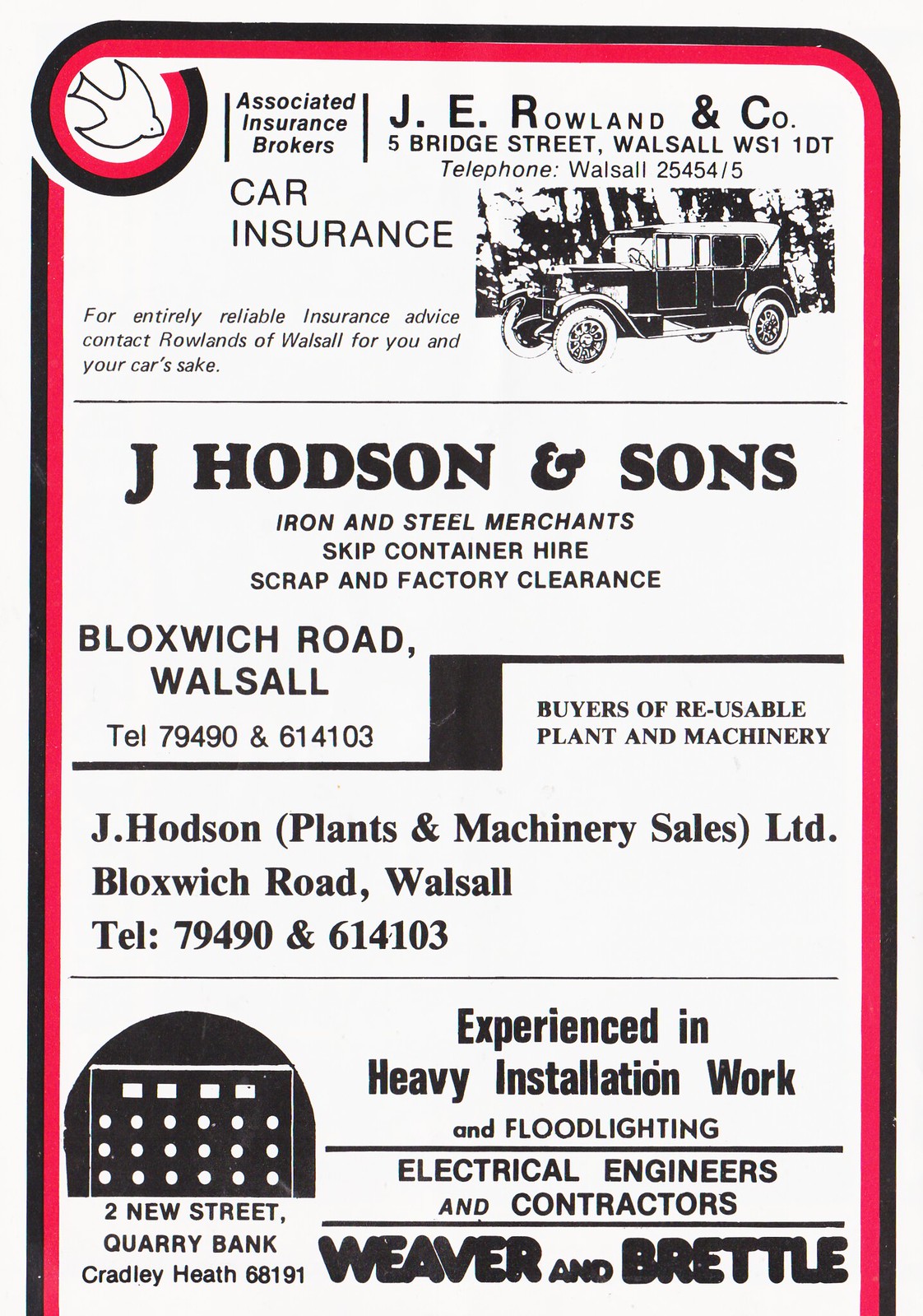This image depicts a rectangular advertisement page from an old magazine, bordered in black and red, featuring a series of black and white ads for various businesses. The top advertisement is for J.E. Rowland & Co., Car Insurance, associated with Insurance Brokers. It includes a detailed contact section with a telephone number and an address, alongside a small illustration of an old-fashioned car with the tagline, "For entirely reliable insurance advice, contact Rowlands of Walsall for you and your car's sake." Below this, in the middle, is a larger ad for J. Hodson & Sons, Iron & Steel Merchants, offering services like skip and container hire, scrap, and factory clearance. Their contact information is clearly displayed, and they also identify as buyers of reusable plant and machinery, operating under the name J. Hodson, Plants & Machinery Sales, Limited. The final advertisement at the bottom promotes Weaver & Brettel, Electrical Engineers & Contractors, experienced in heavy installation work and floodlighting. It presents their street address and includes a small drawing of an office building to the left. Overall, the image showcases an assortment of detailed and vintage-style advertisements, indicative of a bygone era.